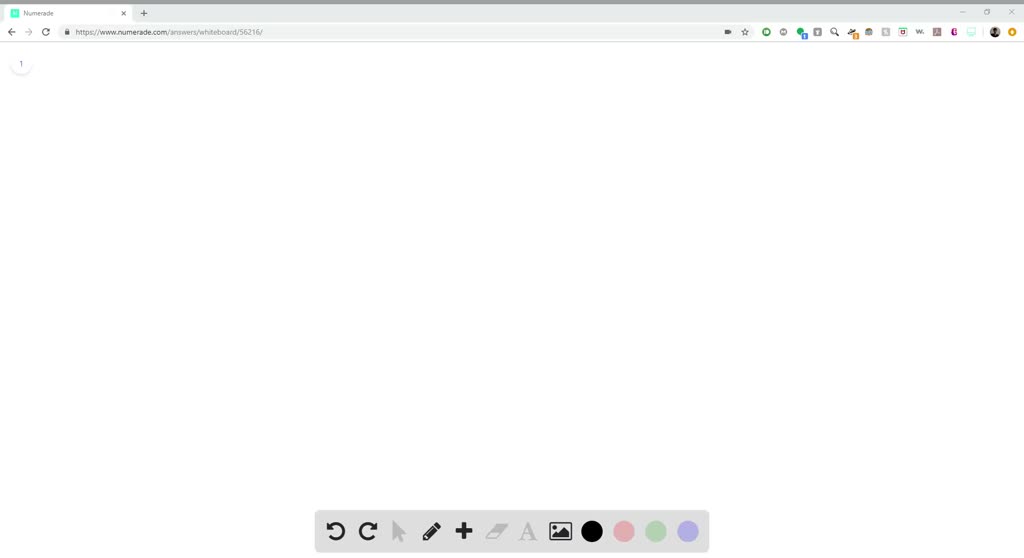The screenshot displays an interface of an online drawing or design tool titled "Numeraid." The screen predominantly features a whiteboard area, on which no content is currently visible, suggesting that it is ready for use or a new session.

In the upper left corner, a small blue or green box reads "Numeraid," alongside a URL: www.numeraid.com/answers/whiteboard. This likely indicates the platform's name and the specific section of the website being used.

The top right corner hosts an array of icons: a star, a green circle possibly linked to notifications, another green circle resembling a Facebook logo, a 'W' icon, a yellow circle with a person silhouette, among others, indicating various tools or shortcuts for user interaction.

At the bottom center of the screenshot, a gray bar spans part of the screen, featuring several icons for editing and drawing functions: a leftward-facing circular arrow (undo), a rightward-facing circular arrow (redo), a pencil or crayon symbol (drawing tool), a black plus symbol (add), a letter 'A' (text tool), and an image icon depicting a mountain (image upload). 

Additionally, there are color dots underneath these tools representing different color options: black, pink, green, and purple circles, suggesting that users can select these colors for drawing or highlighting.

The overall minimalistic and clean design of the interface appears user-friendly, focusing on providing essential tools for creating or editing visual content.